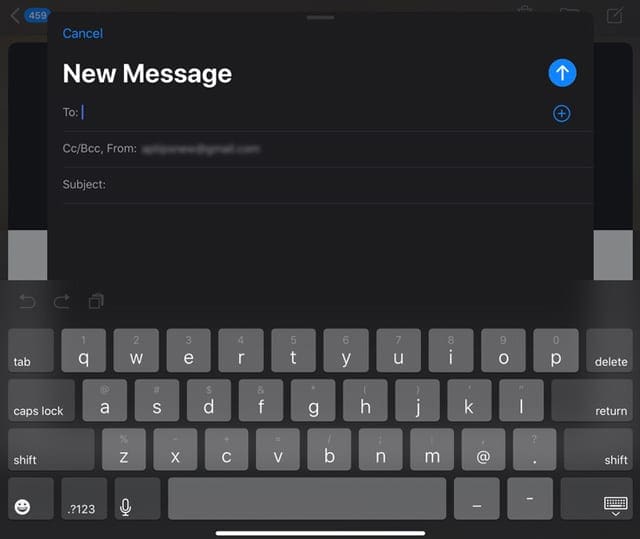A screenshot displays an on-screen interface, likely from a tablet or similar device, featuring an on-screen keyboard. The dark-themed background accentuates various interface elements:

- At the very top, a navigation bar includes a left arrow icon, a blue oval containing the number "459," and a hard-to-see square symbol on the far right.
- Just below, a blue "Cancel" button is on the left, while the title "New Message" is prominently displayed in white in the center, next to a circle enclosing an up arrow.
- The line beneath reads "To:" with a blinking mouse cursor, and a circle with a plus sign is positioned on the far right.
- Following this is the "CC/BCC, From:" field with some text blurred out for privacy.
- The next line contains the "Subject:" field.
- Under these input fields, there are two gray squares on the left and right sides, denoting the message typing area.
- Further down, navigation buttons include back and forward arrows, as well as another square symbol.
- Finally, at the bottom, the detailed QWERTY keyboard layout is shown. It includes keys for tab, caps lock, shift, and a smiley face on the left, and delete, return, shift, and a key to close the keyboard on the right.

This detailed interface layout is indicative of composing a new message on a messaging platform.